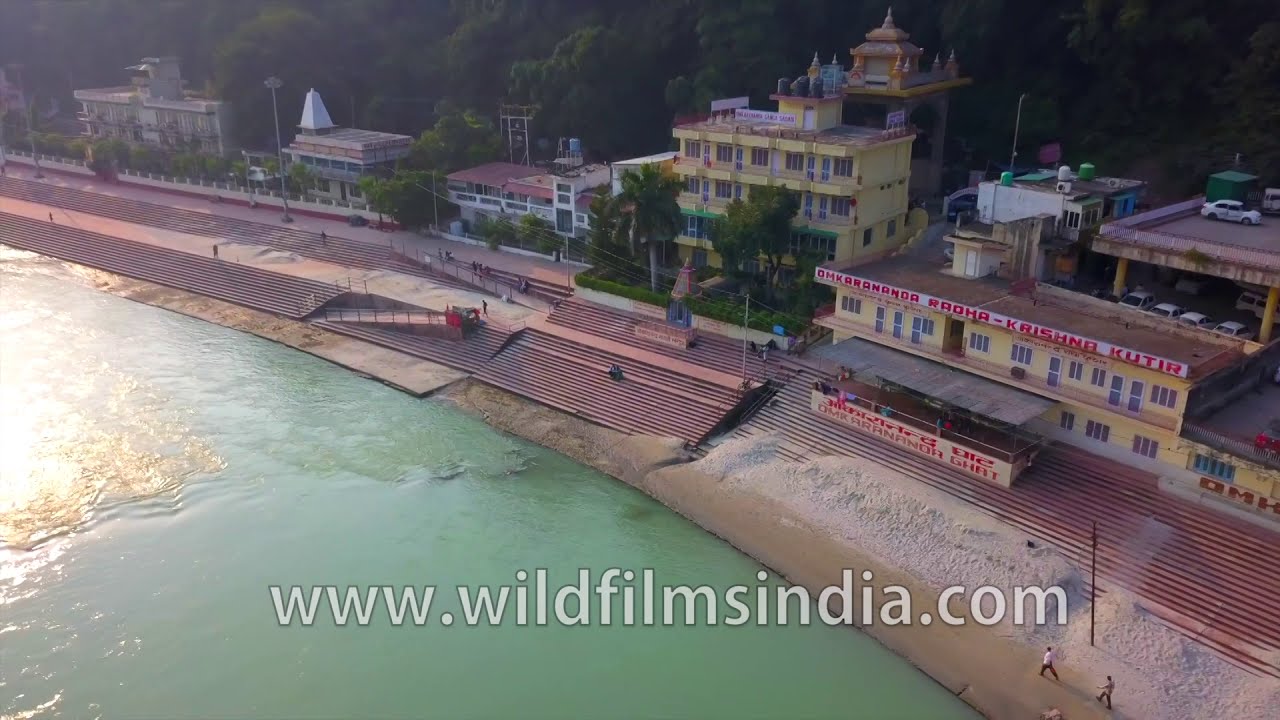This horizontal aerial photograph captures a coastal area in India featuring www.wildfilmsindia.com in white text across the bottom center. The image prominently showcases a body of water to the left, transitioning from calm to slightly rippled. The water is a light green hue. On the right side of the photo, a sandy shore extends upward from the bottom right corner and gradually narrows as it reaches the midsection of the left edge. This shoreline area appears tiled in places, with a thin strip of sand always present to its left. 

Buildings dominate the scene from the lower right corner, extending upward and diagonally to the upper left. These structures vary in height and are predominantly yellow with multi-tiered designs, featuring numerous windows and topped with red inscriptions in an Indian language, hinting at "Kishol Kutur." Stone or possibly red clay stairs lead from the buildings down to the beach. 

Several people are visible along the shoreline and on the steps. In the lower right corner, two individuals walk along a sandy or potentially tiled area, while a couple of others sit on the stairs. More people are seen moving between two stair sets towards the upper left section of the image.

In the backdrop, a dense grove of tall, green trees stretches across the entire top part of the photograph, providing a lush contrast to the vibrant buildings and serene water below. The sunny conditions accentuate the vivid colors and lively atmosphere, evoking a sense of a bustling coastal destination.